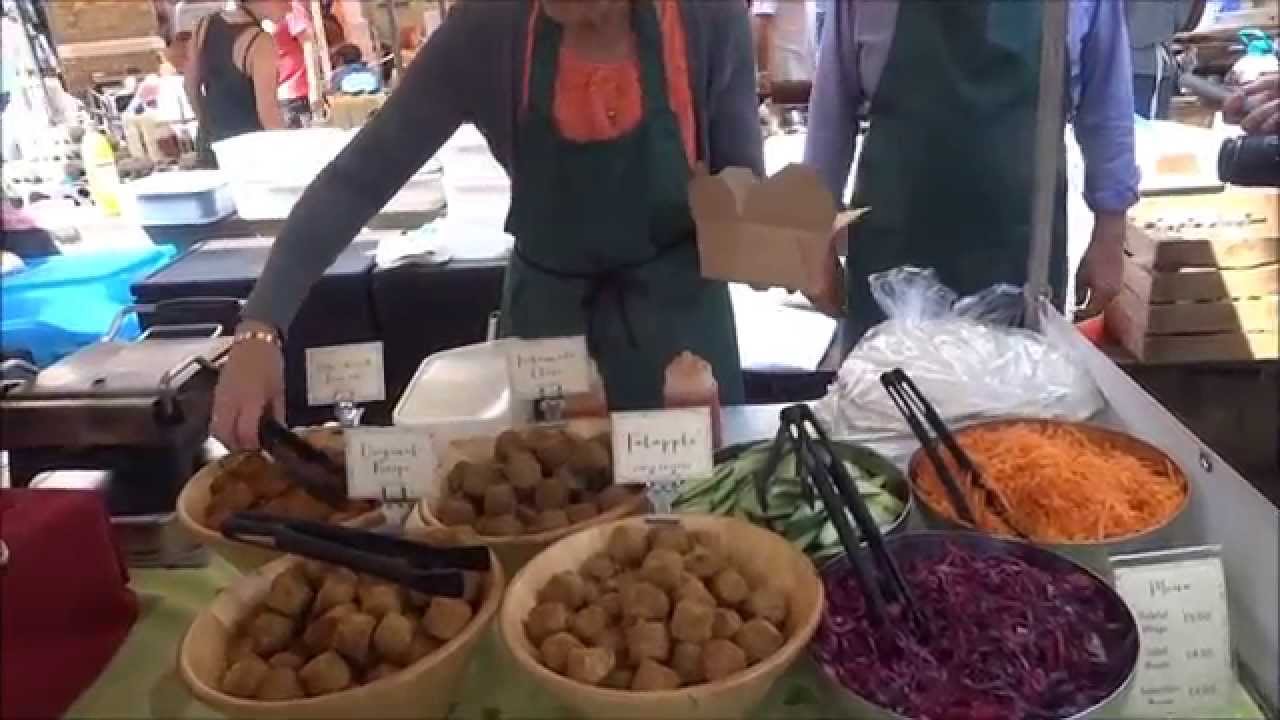This color photograph captures a bustling farmer's market scene, teeming with vibrant vegetables meticulously arranged in bowls, some labeled for convenience. Prominently featured on a green tablecloth-draped table are various vegetables, including shredded orange carrots, purple onions, brown potatoes, and a bowl of green produce. The bowls predominantly exhibit two colors: brown on the left side and silver on the right. Numerous bowls are equipped with black tongs for easy serving.

Situated to the right side of the table is a small, visible price list. The scene is animated by two individuals donning gray aprons. One person, who is wearing an orange shirt underneath their apron, holds a pair of tongs in one hand and a brown box in the other, with a bracelet adorning their arm. The second person, dressed in a long-sleeved blue shirt with rolled-up sleeves beneath their gray apron, is on the left.

The background reveals a sea of activity with other people, illuminated by the shining sun. To the left, stainless steel and black appliances peek through, while a red-covered item and a blue tub of water hint at additional market goods. A woman in the left background sports a daigo with a black bra, striking against a brown wall featuring a white stripe. Scattered across the backdrop are various colored items, such as white and black tubs, and blue, gray, and black boxes, adding to the lively and diverse atmosphere of the farmer’s market.